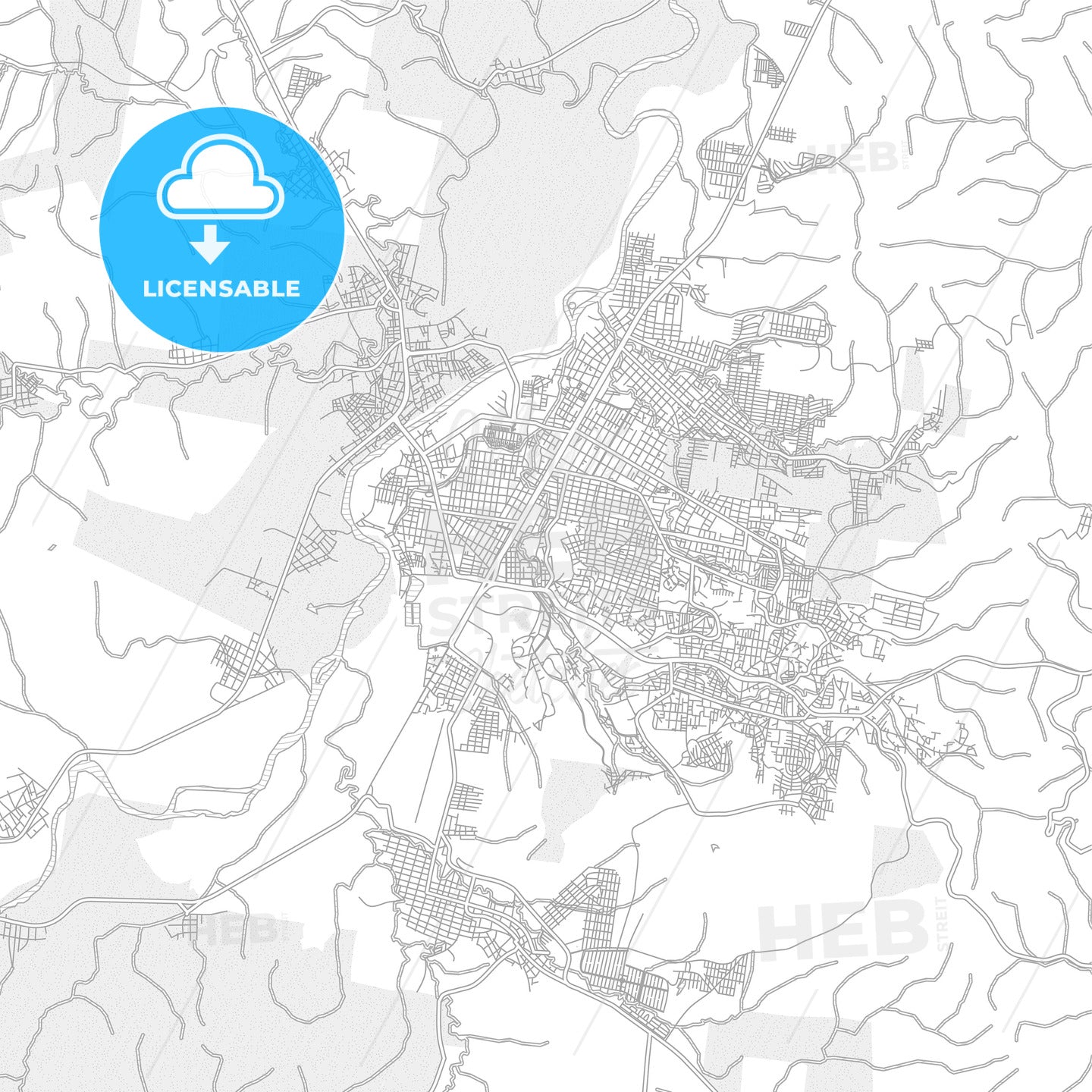The image is a detailed, topographical map of a city layout depicted in black and white. It features tightly packed, intersecting lines indicating densely populated city blocks that gradually disperse as they extend outward from a central river flowing through the middle of the map. The map appears to be hand-drawn or created using CAD software, with precise and clear markers.

In the top left corner, there is a prominent, semi-transparent light blue circle. Inside this circle, a white cloud icon contains a downward-pointing arrow, underneath which the word "LICENSABLE" is written in bold white capital letters. The blue circle is transparent enough to reveal the map details behind it.

Notably, the map does not label streets, buildings, or towns, focusing purely on the geometrical layout of the city. The overall scene is devoid of any color beyond the black and white sketch lines and the distinctive blue marker. Additionally, towards the bottom portion of the map, large semi-transparent letters spell out "H-E-B." The detailed rendering provides a comprehensive view of the city's structure and planning elements.